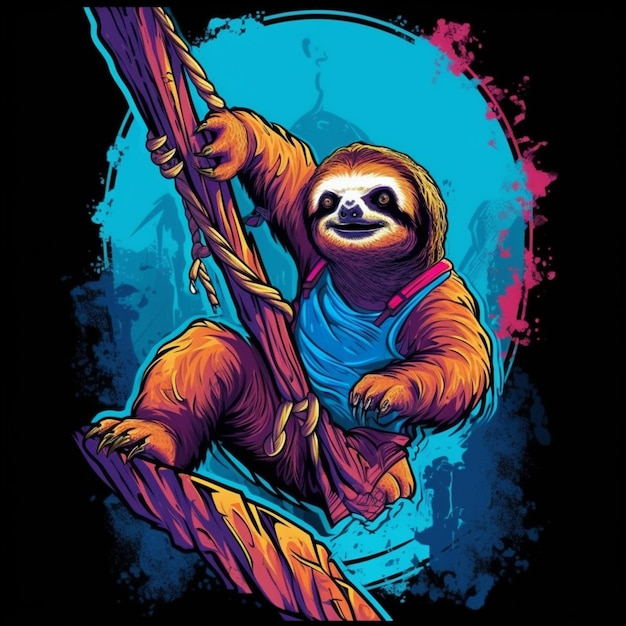The image depicts a detailed, hand-drawn or watercolor painting of a cartoonish sloth set against a black background. Central to the composition is a turquoise-colored, egg-shaped oval outlined in ruby red with magenta blotches scattered along the edges, creating a striking focal point. The sloth, which has brown fur, a white face with black markings resembling a mask around its eyes, a black nose, and a black mouth curved into a smile, is the primary figure. It is personified with human-like features and is dressed in a blue tank top. The sloth is depicted in a playful Tarzan-like pose, hanging and swinging from a grapevine that extends from the left to the bottom of the image. This grapevine is intertwined with a smaller, lighter brown vine. The sloth's limbs are spread out, with its sharp claws gripping the vine, one arm extended out to the side and a leg bent upward, evoking a sense of motion. There is no text present in the image.